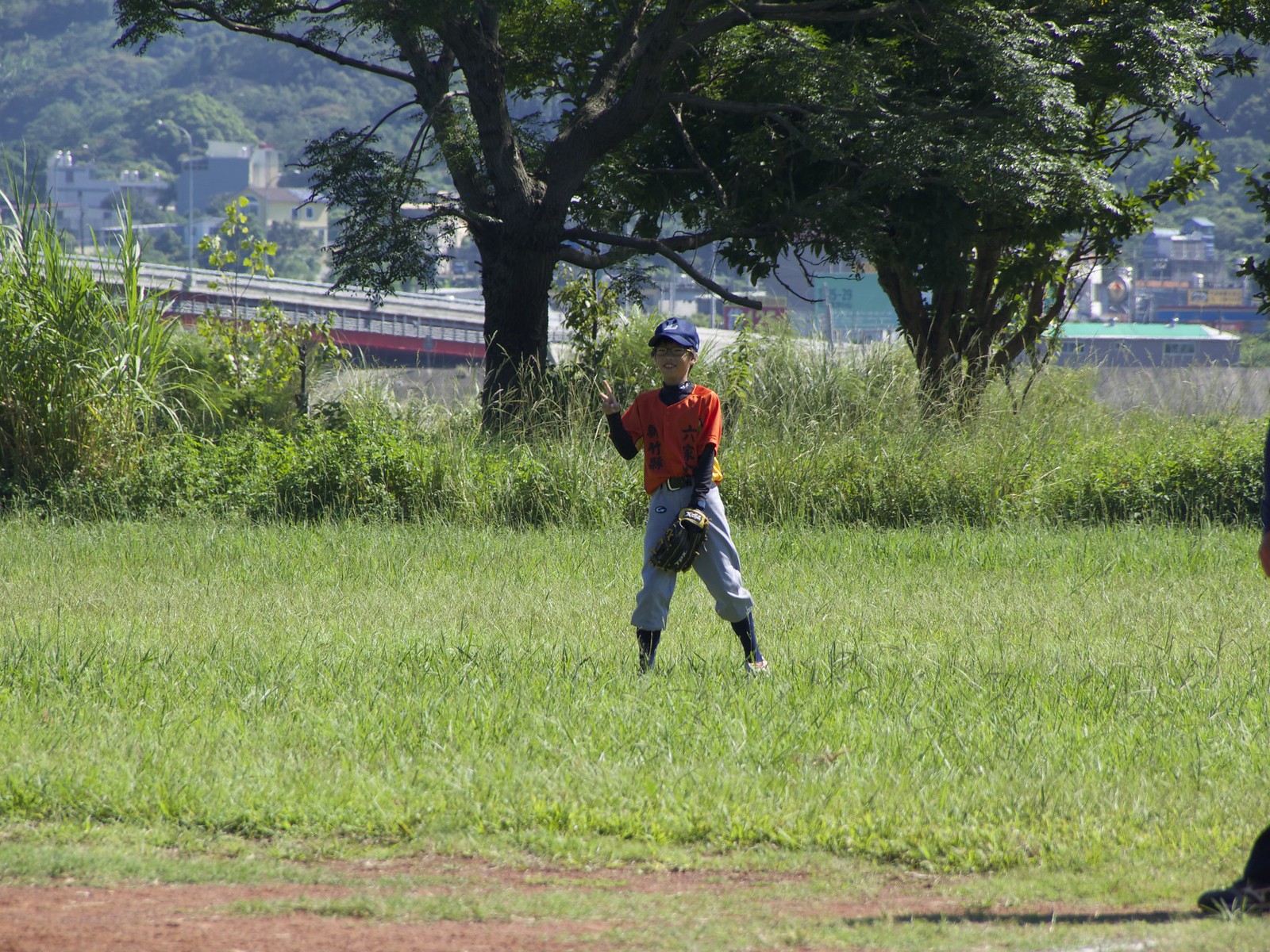This is an outdoor photograph featuring a young boy standing prominently in the middle of a grassy area, dressed in a baseball uniform. The boy is wearing high black socks, sneakers, and gray baseball pants that fall just below his knees. His attire includes a long-sleeve black shirt topped by an orange short-sleeve shirt, and a dark blue ball cap. In his left hand, which is extended downwards between his legs, he holds a black baseball glove, while his right hand is raised, possibly waving or giving a peace sign. 

In the foreground, there is a dirt patch interspersed with grass. Behind the boy, the grassy area transitions into a much taller grass and thick bushes, beyond which stands a large tree with dense green foliage. Further in the background, an overpass or roadway is visible along with several houses and possibly a pool. The scene depicts a bright, clear day, ideal for outdoor activities.